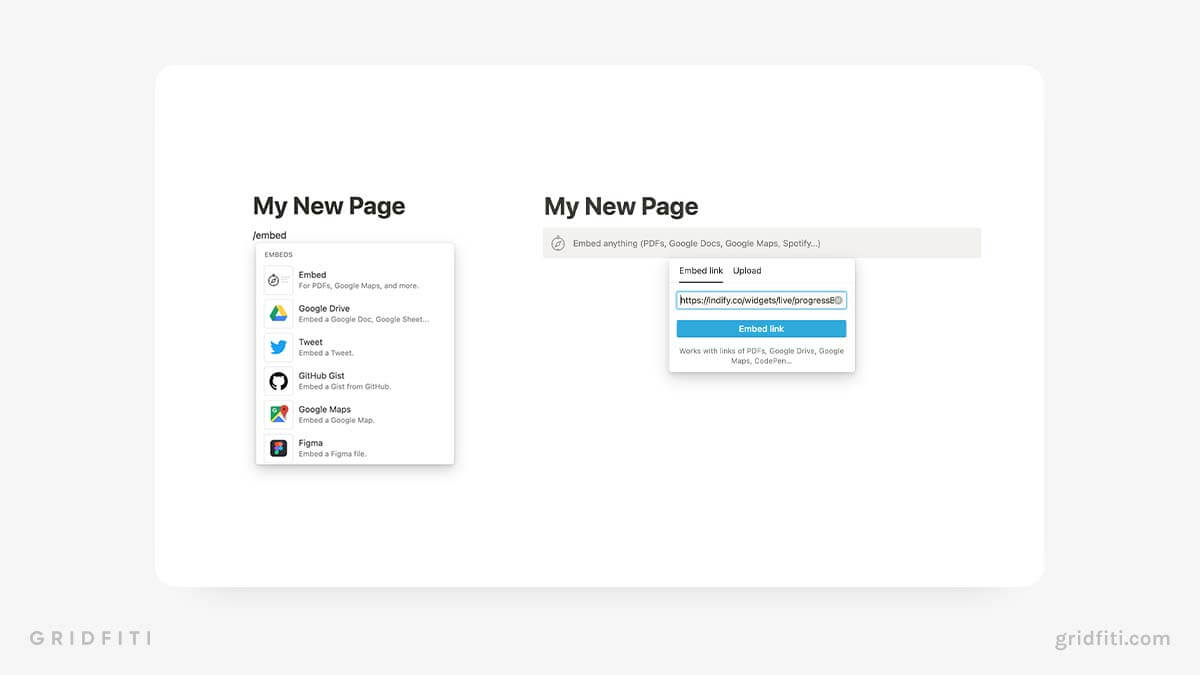This is a detailed screenshot of the Gridfiti website. On the far left, the Gridfiti logo, "GRIDFITI," is displayed in all capital letters with a simple gray font. Above the logo is a line with tapered edges and a subtle drop shadow. 

In the footer, there are two primary sections labeled "My New Page." The left section features a bold header "My New Page" with a slash divider underneath. This section also includes several small icons: a tiny embed icon, Google Drive (a green, yellow, and blue triangle), a Twitter bird icon labeled "Tweet," a GitHub cat icon, a Google Maps icon, and a Figma logo symbolized by the letter "F" in blue and pink.

On the right side, another "My New Page" section is displayed, emphasizing "Embed Anything: PDFs, Google Docs, Google Maps, Spotify." Below this, there are options for "Embed Link" and "Upload" with a field outlined in blue for entering URLs. A large blue button labeled "Embed Link" is visible beneath the URL field. 

The footer also contains links to various menus, including PDFs and Google Drive, although the text is so small (approximately three to four pixels tall) that it is nearly illegible.